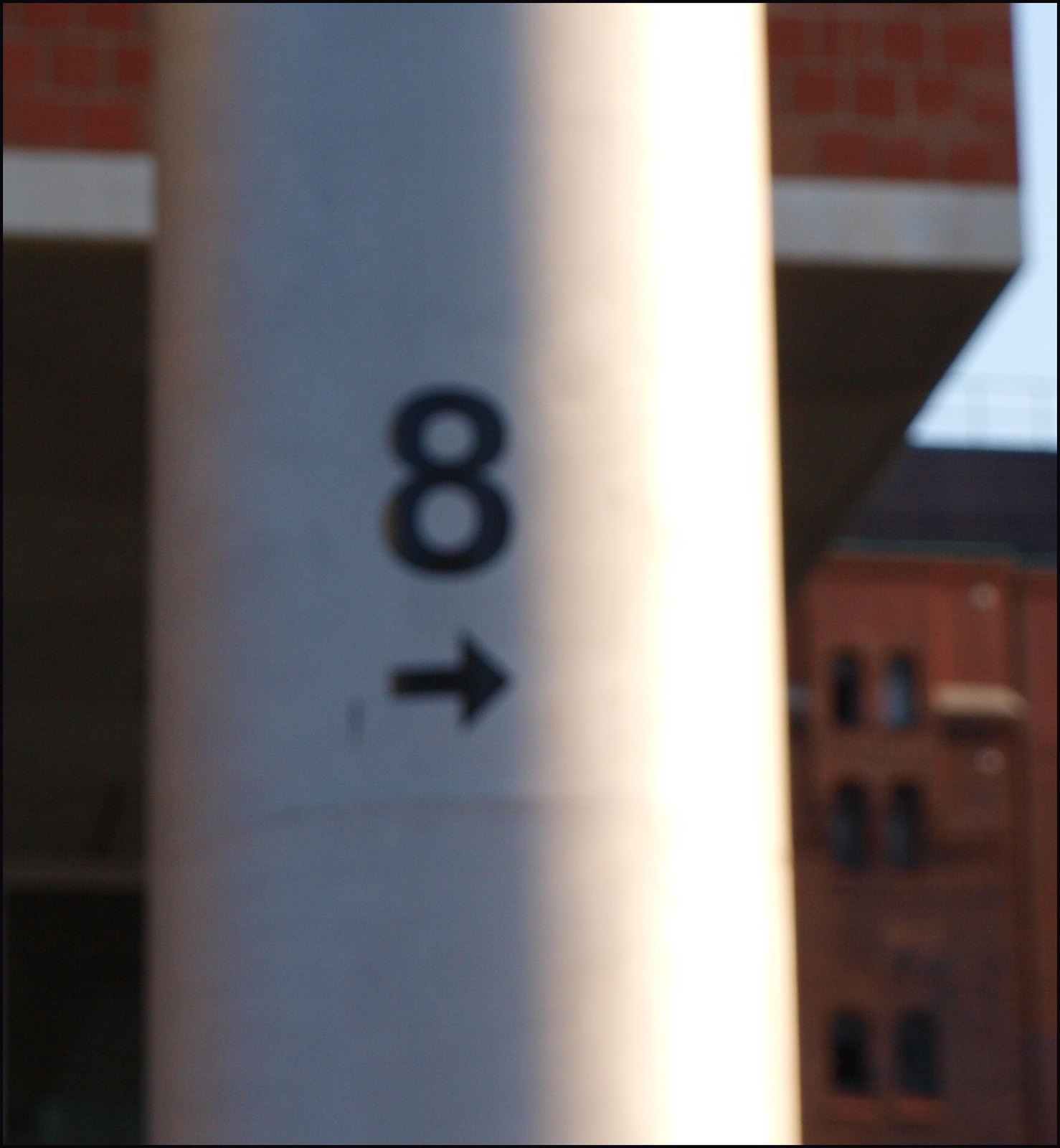The photograph shows a close-up view of a white pole that occupies the center of the image. The pole has a slightly aged appearance and features a prominent black number "8" with a right-pointing black arrow just below it. The pole is partially illuminated by sunlight, casting a shadow halfway across it. In the blurred background, there is a brick building with at least six arch-shaped windows across several stories. Also visible in the background is a red structure with a white stripe at the bottom, angled at about 45 degrees.